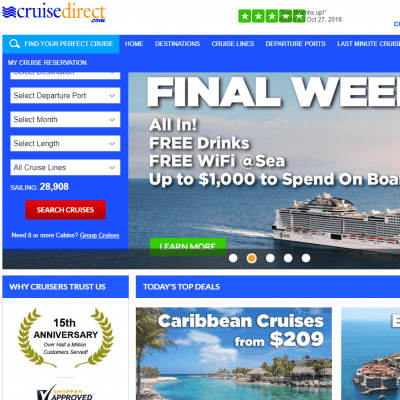Here is a detailed and cleaned-up caption for the screenshot of the CruiseDirect web page:

---

The image depicts a screenshot of the CruiseDirect website. At the top of the page is the CruiseDirect logo, followed by five white stars set against green boxes, indicating rating or quality. Below this section, there is a "Find Your Perfect Cruise" search box that spans the width of the border. To the right of the search box are several darker blue tabs labeled: "Home," "Destinations," "Cruise Lines," "Departure Ports," and "Last Minute Cruise."

Below the search box on the left, there is a section labeled "My Cruise Reservation." Below this are several drop-down menus, including "Select Departure Port," "Select Month," "Select Length," and "All Cruise Lines." A text indicating "Sailing, 28,908" is displayed, followed by a prominent red "Search Cruises" button.

To the right, there's a promotional photograph depicting a sky, a body of water, and a cruise ship. Accompanying the photograph is a banner with the text: "Final Week," "ALL IN! Free Drinks," "Free Wi-Fi at Sea," and "Up to $1,000 to spend on board" (though part of this text is cut off). A "Learn More" link is provided below this banner. 

The webpage also includes a section titled "Why Cruises Trust Us," celebrating their "15th Anniversary Approved" status. On the right side, there is a partially visible section labeled "Today's Top Deals," with an example deal indicating "Caribbean Cruises from $209."

---

This caption gives a structured and detailed description of the content and layout for better understanding and accessibility.